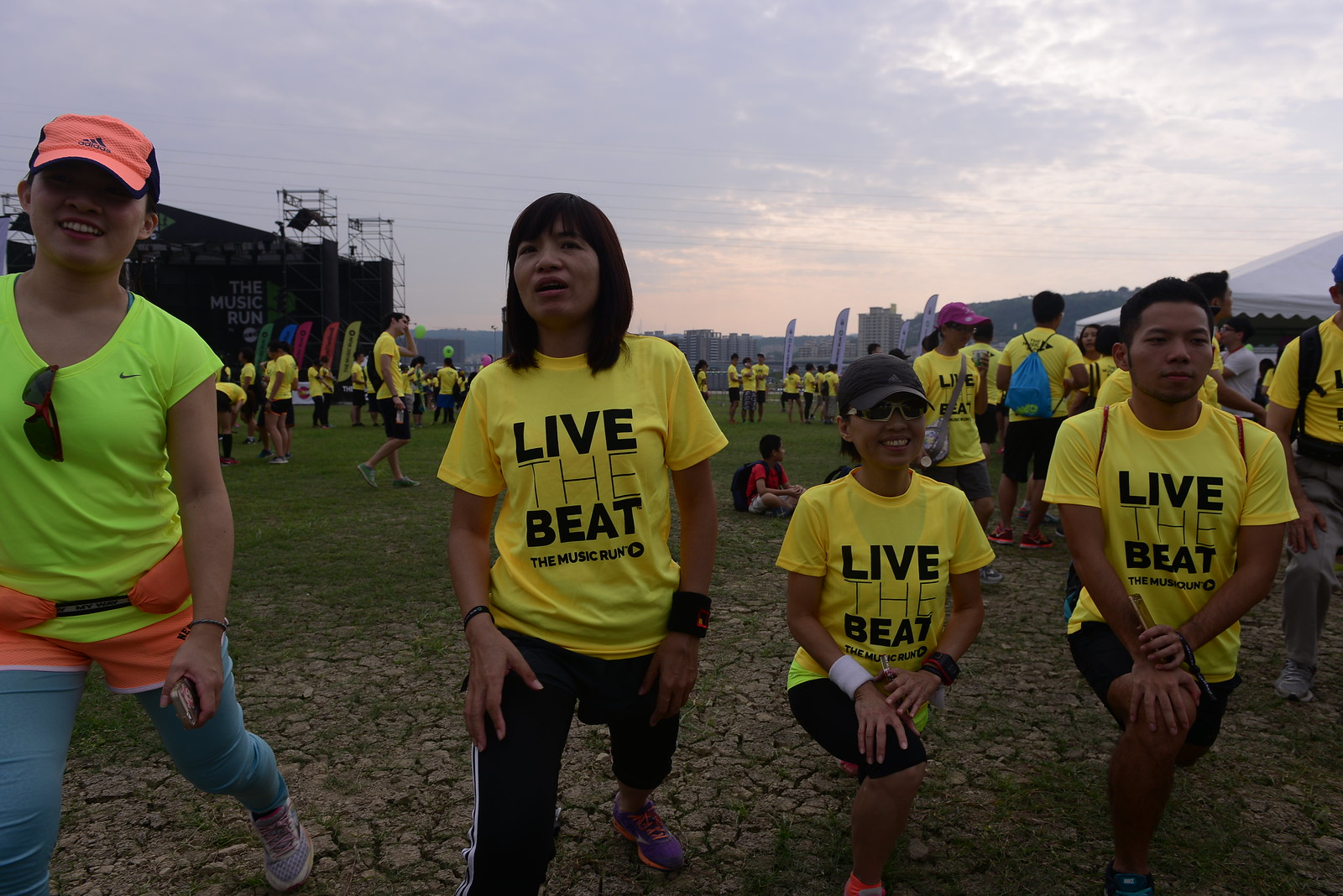The image depicts a bustling outdoor scene, presumably at a music festival gearing up for a race. Dominating the foreground are four individuals, likely of Southeast Asian descent, each performing pre-race stretches. On the left, a woman is outfitted in a lime green Nike shirt, an orange hat, and blue pants with orange shorts layered over them. To her right, three people—two women and one man—are clad in matching yellow shirts emblazoned with "Live the Beat: The Music Run." The woman immediately beside her has black writing on her shirt and wears black pants, while the woman next to her dons sunglasses and a hat. The stretching man at the far right also sports black shorts. The background is teeming with participants, approximately 25 or more, similarly dressed in yellow "Live the Beat" shirts. These individuals are gathered near a prominent stage bearing a banner that reads "The Music Run," hinting at the event's musical theme. The sky overhead is a dramatic mix of gray and orange hues, adding to the scene's lively yet anticipatory atmosphere.